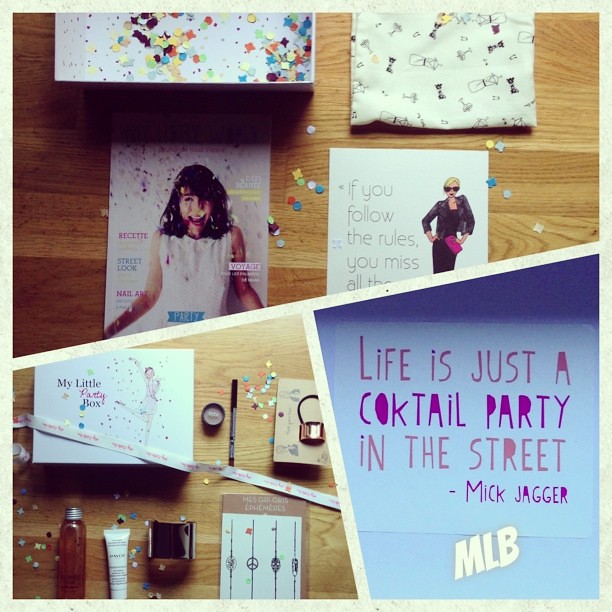The image is a detailed photo collage divided into three sections by white diagonal T-shaped borders. The top section features a brown wood grain surface with four distinct elements: a colorful box of multicolored confetti (red stars, blue circles, yellow stars), a white pillowcase or fabric with various patterns, a beauty magazine cover depicting a smiling woman in a white dress with confetti raining down, and a card that reads, "If you follow the rules, you miss all the fun," accompanied by an illustration of a fashionable blonde woman with sunglasses. The bottom-left section showcases various cosmetic items against the same wood grain background, including a white bottle, clear bottles, a circular makeup container, and a white box labeled "My Little Party Box," illustrated with a dancing woman and a ribbon flowing from the box. The bottom-right section contains a bold text quote in red and purple that reads, "Life is just a cocktail party in the street," attributed to Mick Jagger, with "MLB" noted in white font below.